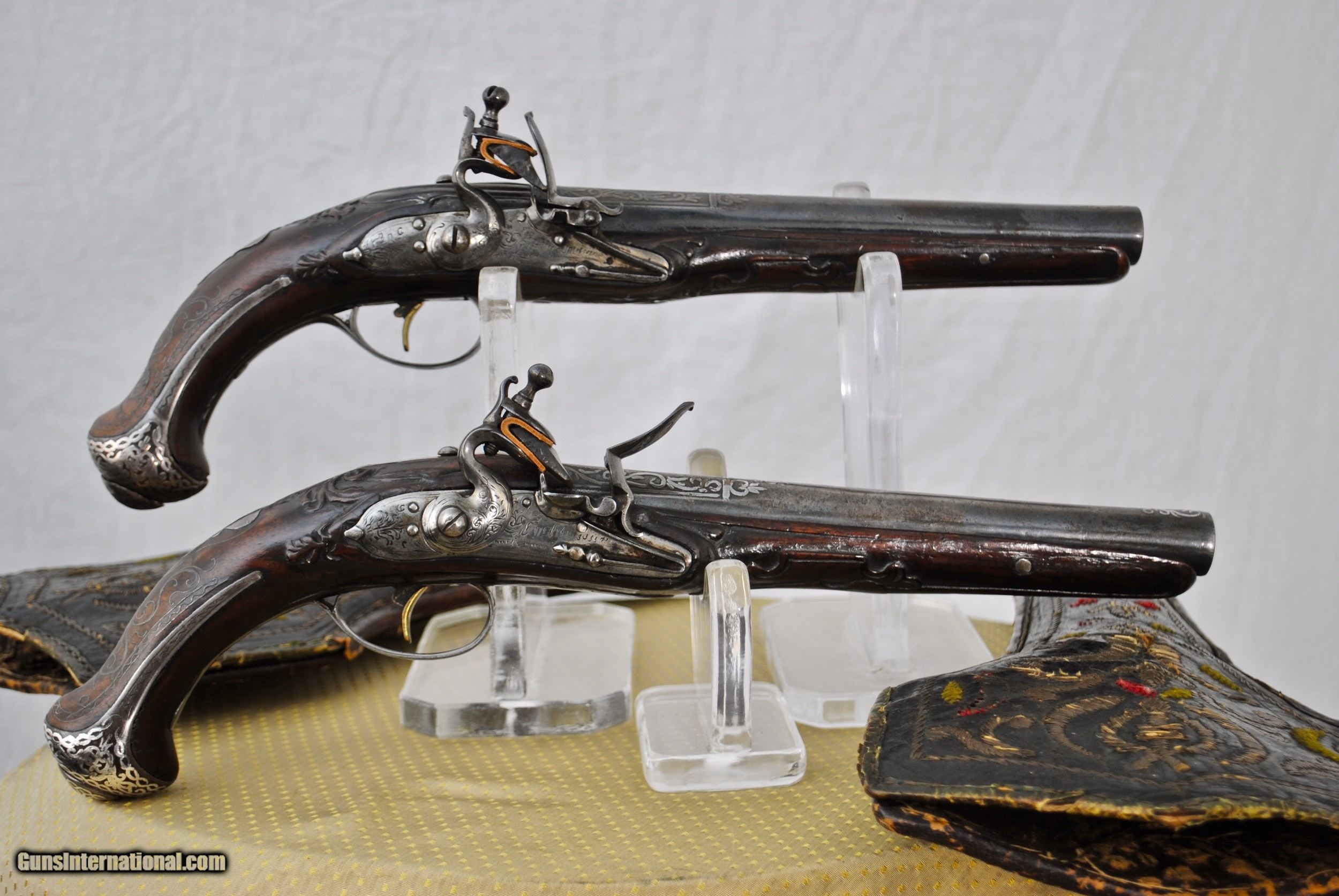This detailed photograph showcases two identical old-fashioned matchlock pistols with intricately designed handles and barrels. The pistols’ handles are carved from what appears to be deep mahogany wood, elegantly finished with silver details, including a buttplate to prevent scratching. The curved handle and underbarrel form a single piece, making the pistols easier to grip. The black metal barrels and mechanisms are prominently featured, with the pull-back mechanism located atop the pistols rather than near the trigger. Both pistols rest on clear acrylic stands, positioned on a round table covered with a yellow tablecloth. Additional artifacts resembling painted wooden items, potentially shaped like bicycle seats, are also displayed on the table. The photograph is set against a white cloth background with a visible watermark, "gunsinternational.com," at the bottom left corner.